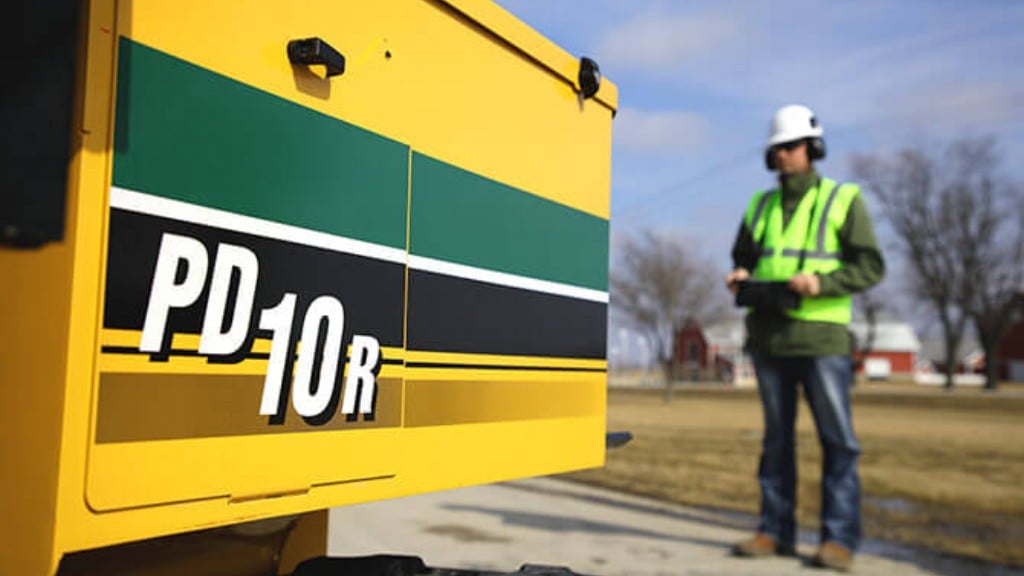The photograph captures an outdoor construction scene on a bright, sunny day, with a mix of detailed and blurred elements. The left side prominently features a yellow rectangular piece of equipment adorned with stripes: green, black, a smaller white stripe, a tiny black stripe, and a dark yellow stripe. The equipment is marked with the text "PD10R" in white letters, and a black handle is visible above the stripes. 

On the right side of the image stands a construction worker on a gray roadway. He is wearing a white safety helmet, black ear defenders, sunglasses, a long-sleeved olive green shirt, blue jeans, brown hiking boots, and a light green reflective safety vest. He appears to be holding a clipboard or tablet. 

In the blurred background behind him, there is a red and white house, brown grass, bare trees, and a field area under a blue sky dotted with scattered white and fluffy gray clouds. The photograph blends precision in the equipment's details with a broader, slightly unfocused depiction of the environment and the worker.